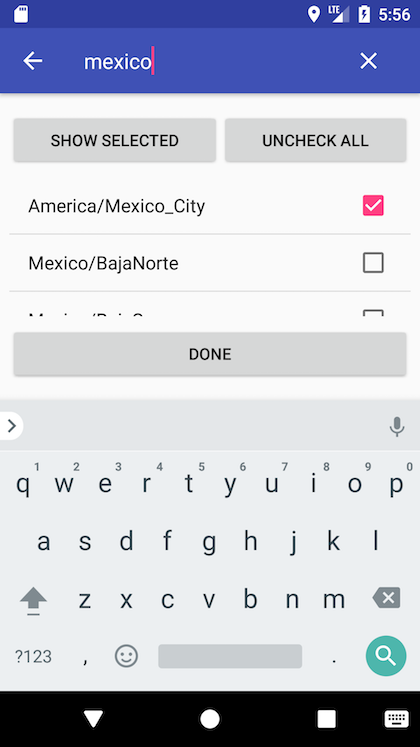This is a detailed view of a cell phone screen. At the very top, there is a blue strip, slightly darker, housing all the standard cell phone icons. On the right side, you can see a location pin icon, cell phone signal bars, and a battery icon that shows a charge level of 56%.

Below this strip, there is a navigation bar with a left-facing arrow labeled "Mexico" and a red line following it. To the right of "Mexico" is an X icon. Directly under this bar, two grey buttons with black text read "Show selected" and "Uncheck all."

In the main content area, the text "Americana/America/Mexico_city" is displayed, accompanied by a checkbox on the right that is filled in red with a white checkmark. Below that text is "Mexico/Baja Norte" with an outlined checkbox that is not selected. Another option exists below, but it is not visible in the image.

Towards the bottom, a long horizontal button labeled "Done" can be seen, featuring grey background and black text. Below this button, the virtual keyboard is pulled up, predominantly grey with black letters; the individual keys are not distinguishable, just the letters.

At the very bottom, a black strip hosts several white icons including a down arrow, a circle, a square, and a keyboard icon.